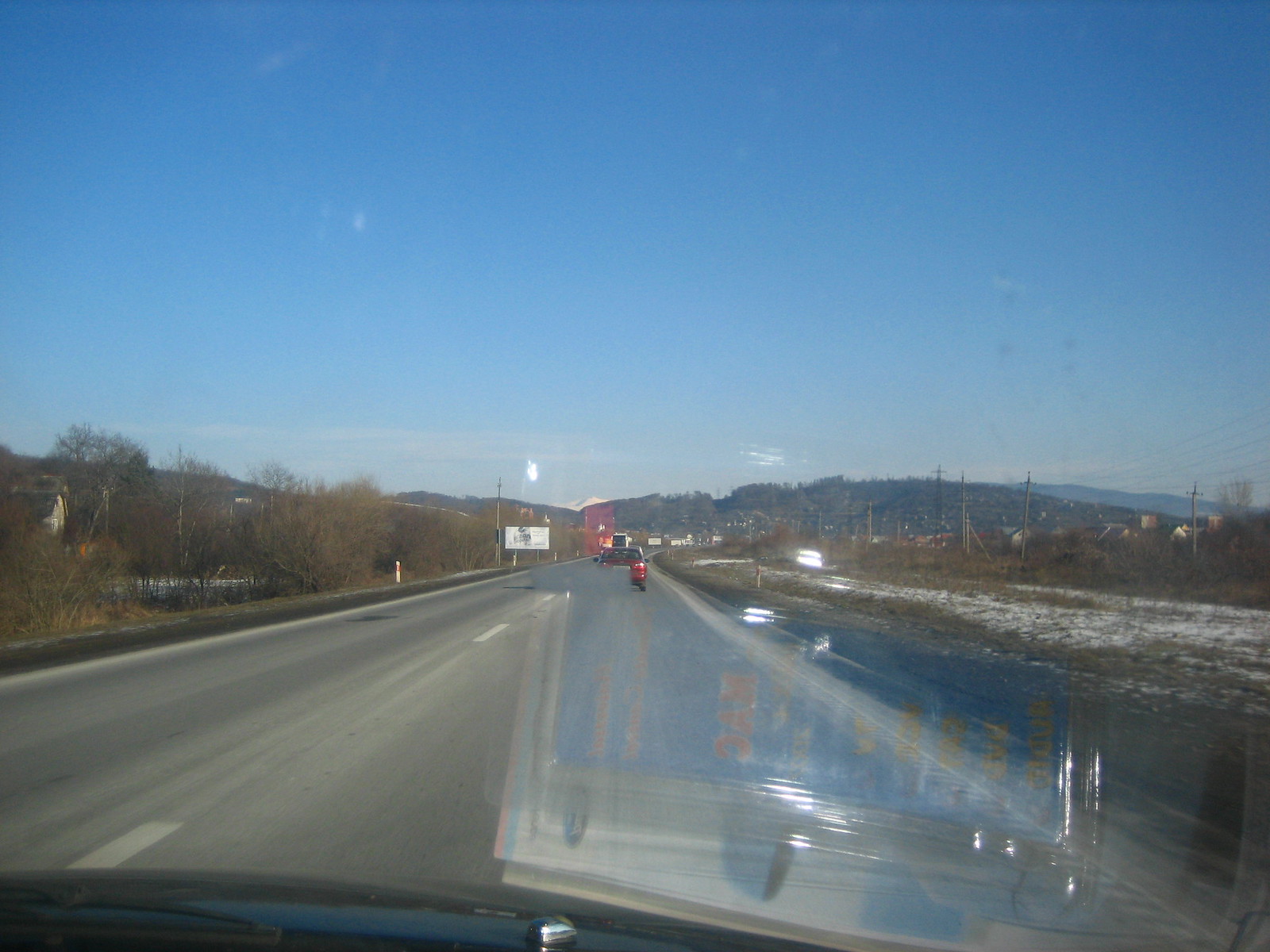The image depicts a two-lane highway during winter, captured from the front passenger seat of a vehicle. The setting is a mostly clear, blue sky that transitions from a vibrant medium blue at the top to a light blue at the horizon. In the distance are tree-covered hills and a few mountains. Alongside the road, there are dormant or dead plants, with some trees and bushes scattered about, as well as power lines extending into the distance. 

On the left side of the road, there's a small, white billboard. Directly in the vehicle's lane ahead, there's a red Vespa or small red vehicle, and in the other lane, farther ahead, there appears to be a white truck or possibly a combine harvester or tractor. The photo distinctly captures a reflection of a blue and yellow license plate or a blue rectangular item on the windshield, and there is a faint view of the car's dashboard.